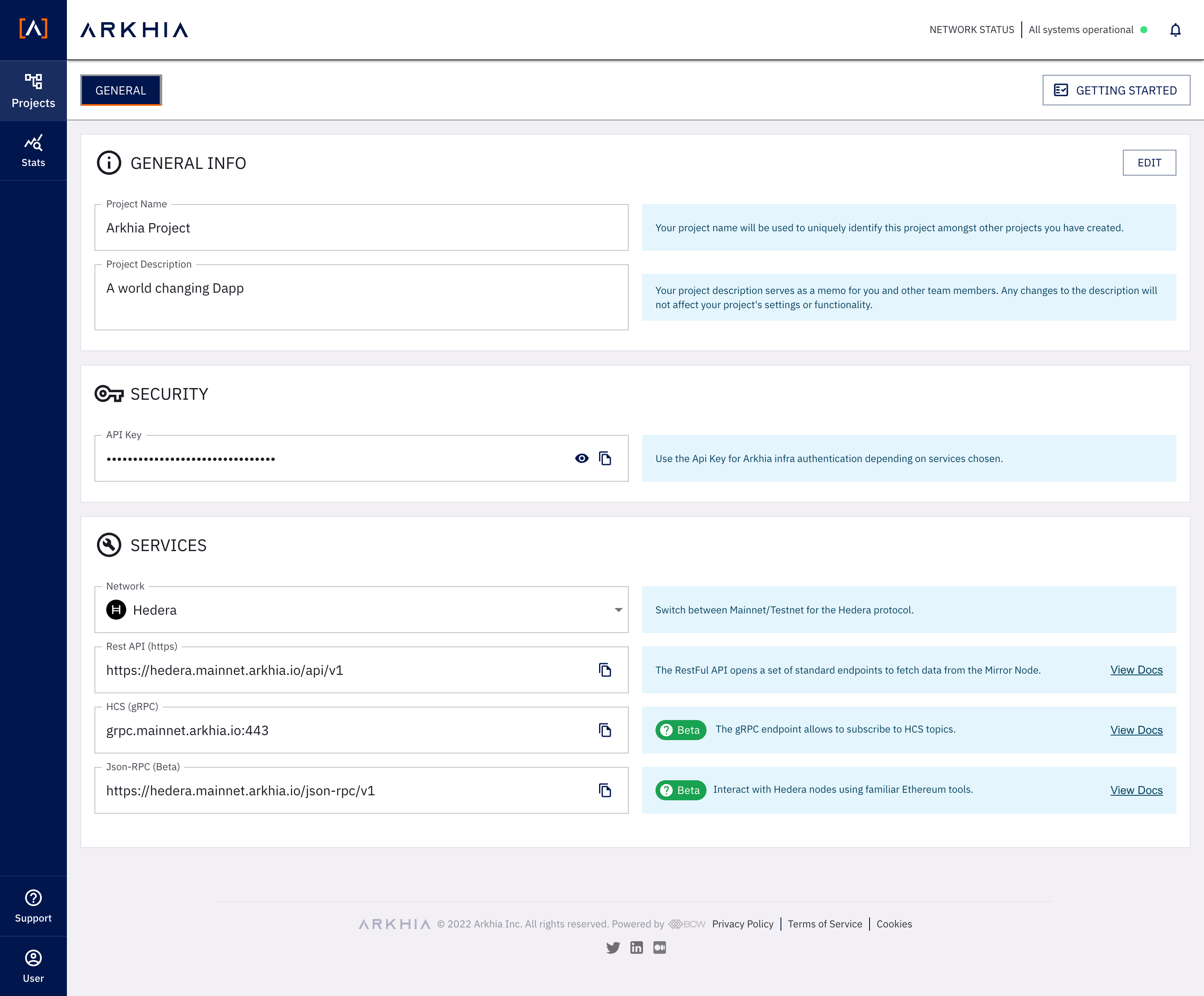Screenshot of Arcea Website

The screenshot captures various sections and elements of the Arcea website interface. At the top left corner of the screen, the "Arcea" logo is prominently displayed. Directly beneath the logo, there is a blue "General" button. Running vertically along the far left side of the screen is a navy blue stripe. At the top of this stripe is an "A" encased within two orange brackets. Below this are icons for "Projects" and "Stats," separated by a considerable gap from the icons for "Support" and "User," which are located at the bottom left side.

The main page of the screenshot features three distinct sections organized into separate white boxes: "General Info", "Security", and "Services". Each white box has input fields on the left side for users to type in information and a light blue banner on the right side providing explanatory text for each section or row.

1. **General Info:**
   - **Project Name:** Arcea Project
   - **Project Description:** A world-changing DAPP
   - At the top right of this box, there is an "Edit" button, and above the box, there is a "Getting Started" button.

2. **Security:**
   - **API Key:** The key is redacted and accompanied by an eye icon that allows users to toggle the visibility of the key.

3. **Services (comprising four rows):**
   - **Network:** Information provided with a relevant web address.
   - **Hedera:** Information provided with a relevant web address.
   - **REST API:** Contains a web address along with an eye icon and a "View Docs" link.
   - **HCS:** Contains a web address along with a green "Beta" button and a "View Docs" link.
   - **JSON RPC:** Contains a web address along with a green "Beta" button and a "View Docs" link.

Overall, the screenshot provides a comprehensive overview of the essential interface elements and functionalities available on the Arcea website, focusing on project information, security settings, and service connections.